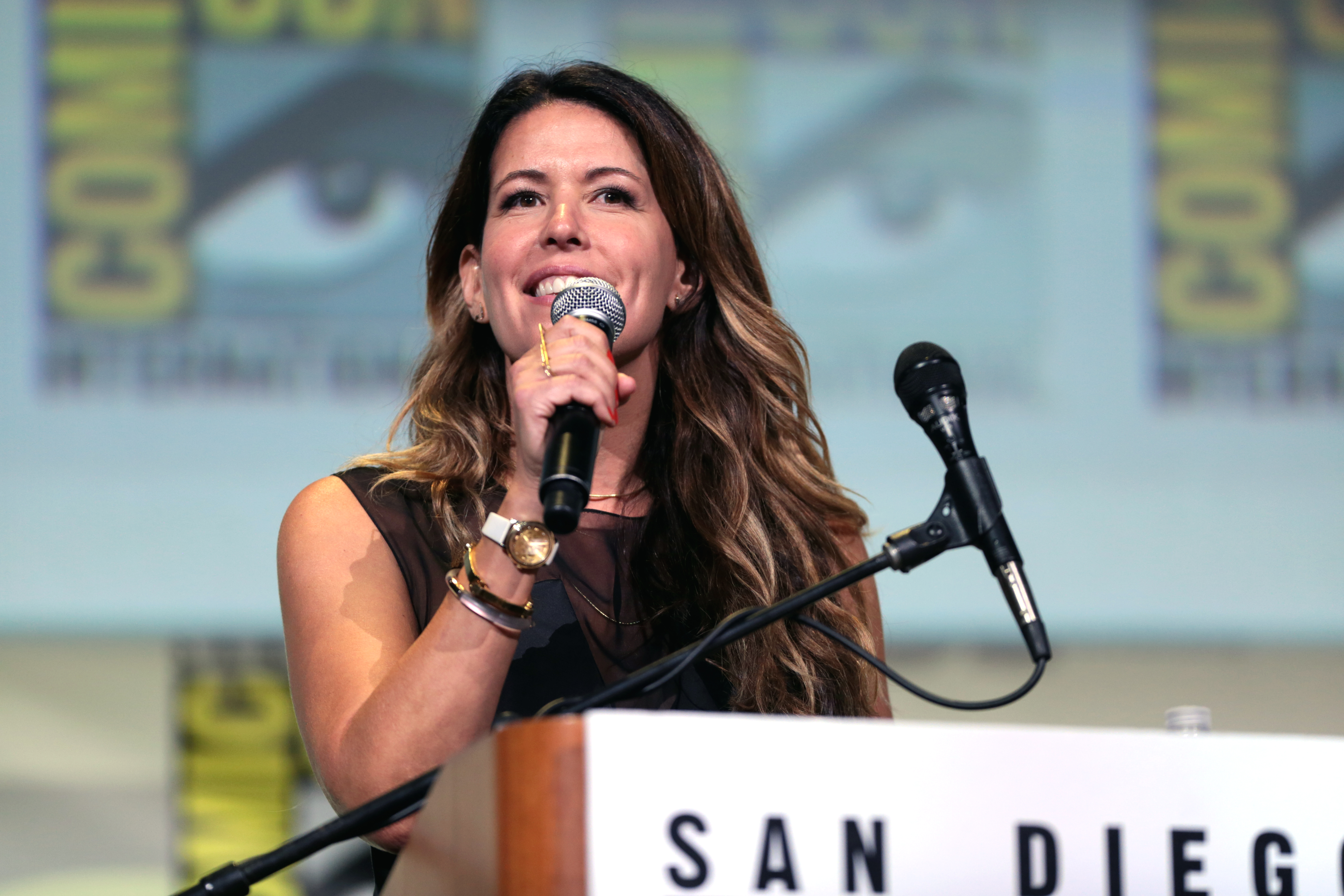The photograph captures a moment at the San Diego Comic-Con. Central to the image is a Caucasian woman with long, dirty blonde, wavy hair that has some blonde highlights. She is standing at a wooden podium with a white sign that reads "San Diego" in black uppercase letters. The woman is dressed in a black cap sleeve shirt that appears slightly transparent towards the upper chest, and she's adorned with a wristwatch and a couple of gold bangles on her right arm. She is smiling and appears to be speaking into a silver-topped microphone that she holds close to her face. Another microphone, mostly black with a bit of silver at the bottom, is positioned diagonally on a stand in front of her. Behind her, three square posters are arranged horizontally on a light blue background. The posters, which appear to feature comic-style artwork, spell out "COMIC-CON" in bold uppercase yellow letters, with "COMIC" running vertically on the left and "CON" across the top. The posters in the center are slightly more blurry than those on the sides. The scene suggests she's engaged with the audience, perhaps answering questions or delivering a talk.